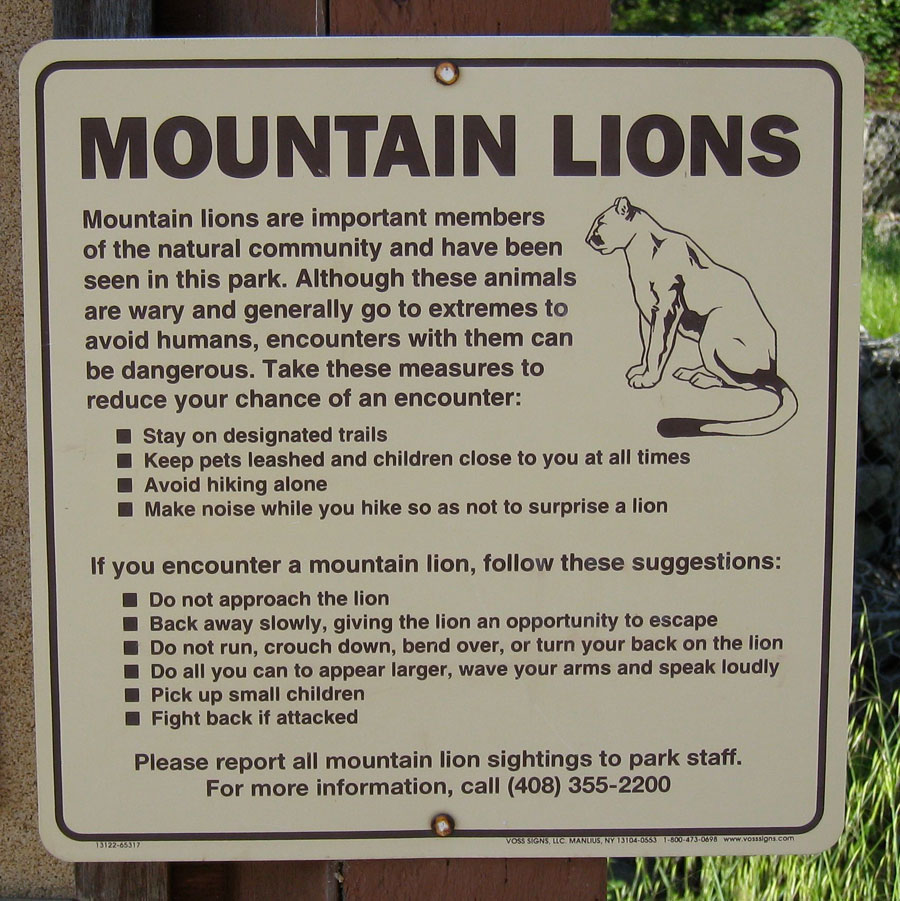This outdoor image captures a detailed sign posted on a white wooden post with a brown base. The sign stands in a park, with grass and a rock wall visible in the background. The sign's top prominently displays the bold words "Mountain Lions," accompanied by a black-outline drawing of a mountain lion sitting with its tail wrapped around its front, gazing left. The sign's background is a beige color with a black border, giving it a clear and formal appearance.

The text emphasizes that mountain lions are crucial members of the natural community and have been seen in the park. While these animals usually avoid humans, encounters can still be dangerous. To reduce the chances of encountering a mountain lion, visitors are advised to stay on designated trails, keep pets leashed and children close, avoid hiking alone, and make noise while hiking to avoid surprising a lion.

If an encounter occurs, the sign suggests specific actions: do not approach the lion, back away slowly to allow the lion to escape, avoid running or turning your back, make yourself appear larger by waving arms and speaking loudly, pick up small children, and be prepared to fight back if attacked.

Finally, the sign asks visitors to report all mountain lion sightings to park staff and provides a contact number for more information: 408-355-2200.